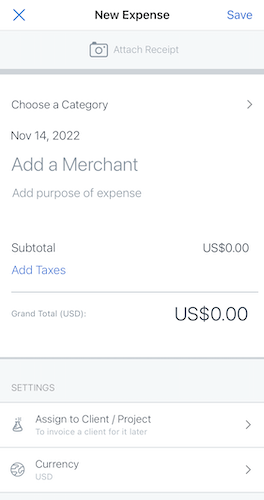The image depicts an interface for recording a new expense. In the upper left-hand corner, there is a blue "X" icon. Prominently displayed in black bold letters are the words "New Expense." The "Save" button is grayed out but highlighted in blue. Below, a gray rectangular box features a camera icon and the text "Attach Receipt." A thick gray line separates this section from the one beneath.

In the next section, the text "Choose a Category" appears, accompanied by a right-facing arrow. The date "November 14, 2022" is displayed. The interface then prompts the user to "Add a Merchant" in very large letters. Underneath this, the statement "Add Purpose of Expense" is shown in gray.

Further down, the interface lists "Subtotal" with the amount displayed as "USD 0.00." There is an option to "Add Taxes" highlighted in blue, but this feature is currently grayed out. Another gray line comes next, followed by "Grand Total (USD):" with the amount "USD 0.00" shown in large letters.

At the bottom, a gray bar is present with a lighter gray rectangle containing the word "SETTINGS" in all capital letters. Below this, there is an icon resembling a flask along with the text "Assign to Client/Project" and, in smaller letters, "to invoice a client for later," accompanied by a right-facing arrow. Another icon, a globe, indicates the "Currency" as "USD," also with a right-facing arrow.